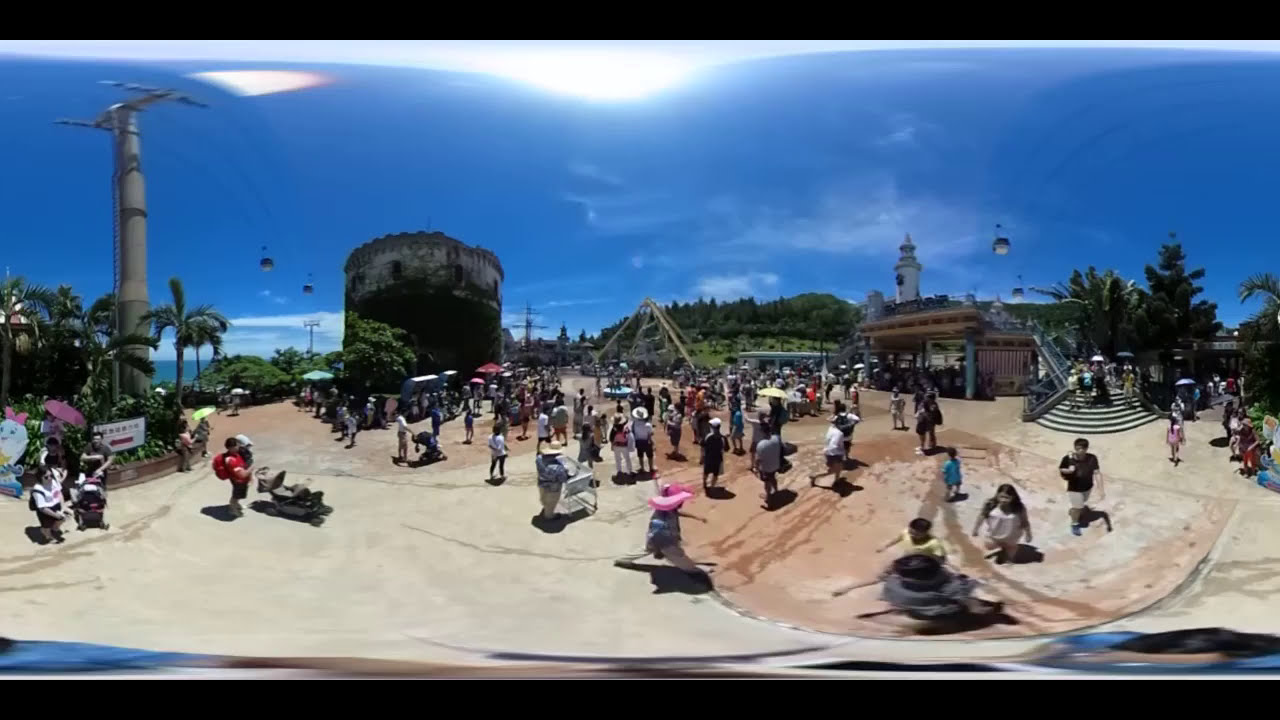This photograph, likely captured using a fisheye lens, presents a sweeping view of a bustling outdoor tourist area set in a tropical climate. The scene is illuminated by the sun under a vibrant blue sky with a few wispy clouds. Central to the image is a large, white and brown ground, populated by numerous people enjoying the pleasant weather. Some people, equipped with sun hats and umbrellas, are walking around or pushing strollers, highlighting the day's heat.

Dominating the landscape are notable architectural structures. On the right, a historic cylindrical castle stands out, with its black lower walls and white upper walls showing signs of age. A nearby building features stairs crowded with visitors. To the left, there's a gondola-like ski lift system, with towers supporting the wires and small cars visible in the distance, adding a modern touch to the historical setting.

The edges of the scene reveal natural elements, including scattered palm trees and a distant dirt hill adorned with trees. The ocean is faintly visible on the left, adding to the serene backdrop. Additionally, a tower in the center-right, possibly with a clock face, rises above the picturesque scenery, completing the diverse and vibrant portrayal of this tropical tourist destination.